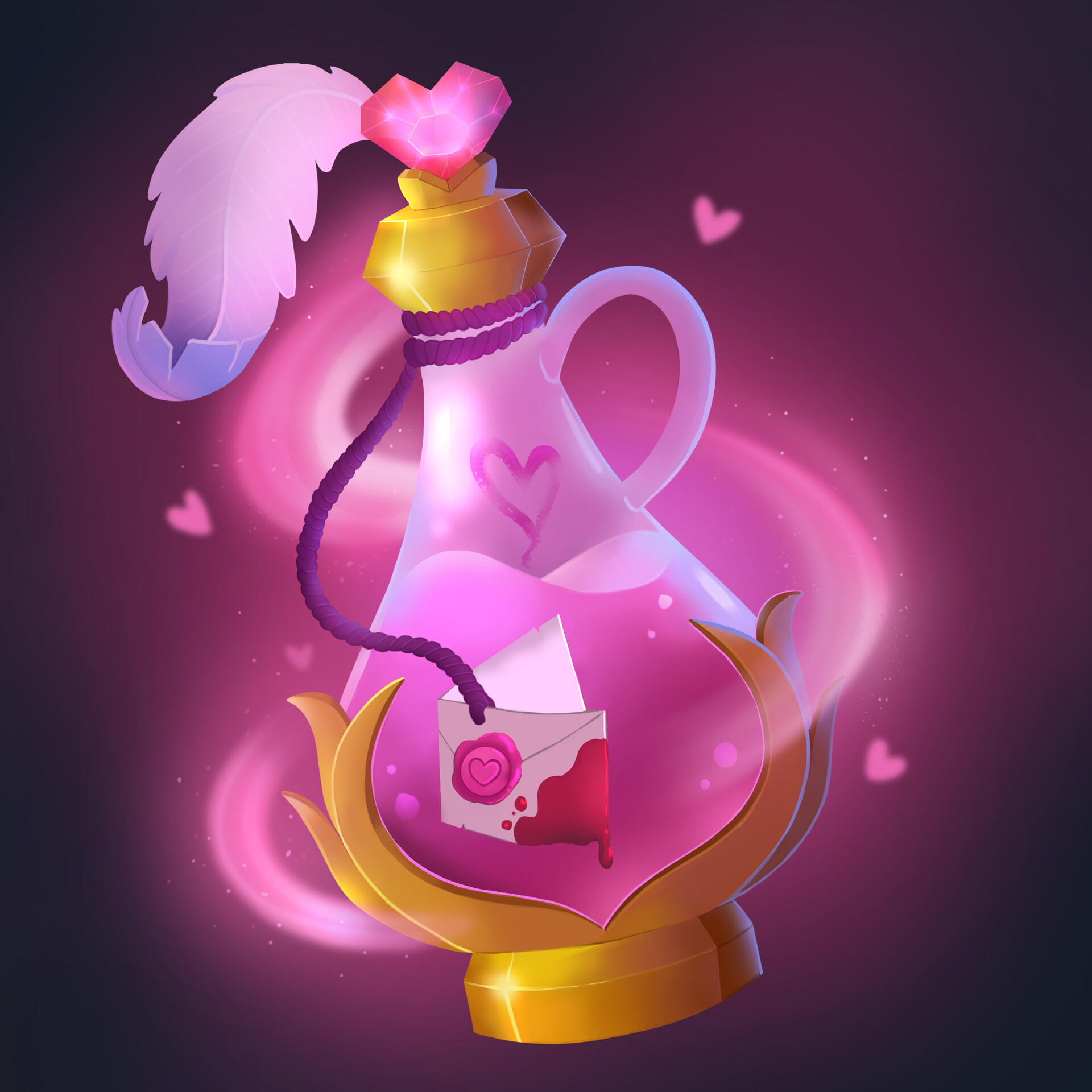The image depicts a whimsical, cartoon-style potion bottle set against a nearly black, dark purple background. The large, clear glass bottle is filled with a pink potion that bubbles inside. The bottle itself is designed in a fantasy genie style, featuring a golden base that curls decoratively around the glass and a matching golden stopper. Adorning the top of the bottle is a fluffy pink feather that elegantly curls at the end. Also, part of the stopper includes a braided purple ribbon tied to an envelope sealed with a bright pink wax heart. The envelope's corner is dipped in a dark red substance, possibly blood or wax, which drips within the potion. Additional details include hand-drawn pink hearts on the neck of the bottle and three floating pink hearts around it. A swirl of pink smoke encircles the bottle, enhancing its magical aura.